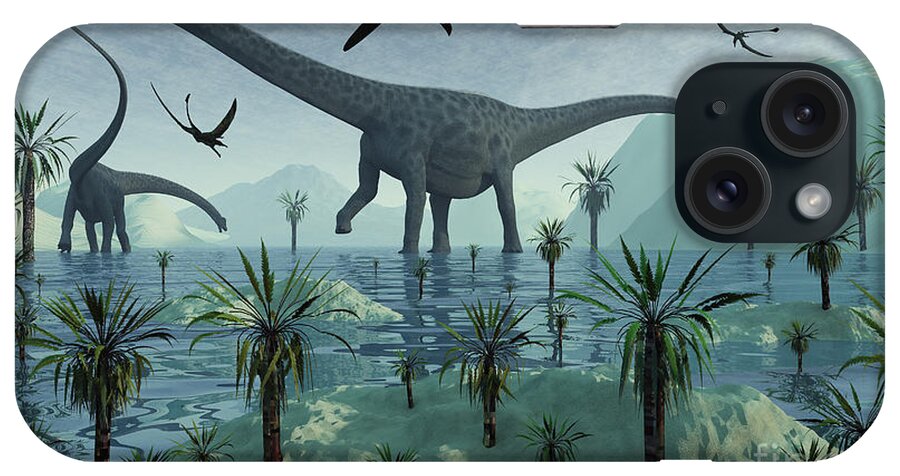The image depicts a horizontally oriented iPhone, possibly an iPhone 13, showcasing a distinctive phone case covered with a detailed color illustration of a prehistoric scene. The phone case features a vibrant and lush depiction of several dinosaur species amidst a water-filled basin bordered by mountains. Central to the scene are two massive sauropods, likely brontosauruses or Argentinosauruses, with sinuous necks and long tails, wading through deep blue water. One of the dinosaurs is centrally positioned but partially obscured by the phone's dual diagonal cameras situated in the top right corner. The tail of this dinosaur extends towards the top left of the phone case, while another fully visible sauropod is bowing down on the left side. Surrounding the dinosaurs are flying pterodactyls soaring through a sky dotted with proto-palm trees and small patches of land protruding from the water. The phone's background is predominantly blue and green hues, imparting a vibrant yet tranquil prehistoric swamp-like atmosphere. The case combines artistic illustration with possibly AI-assisted design elements, covering the phone’s back entirely and standing out against a plain white backdrop.